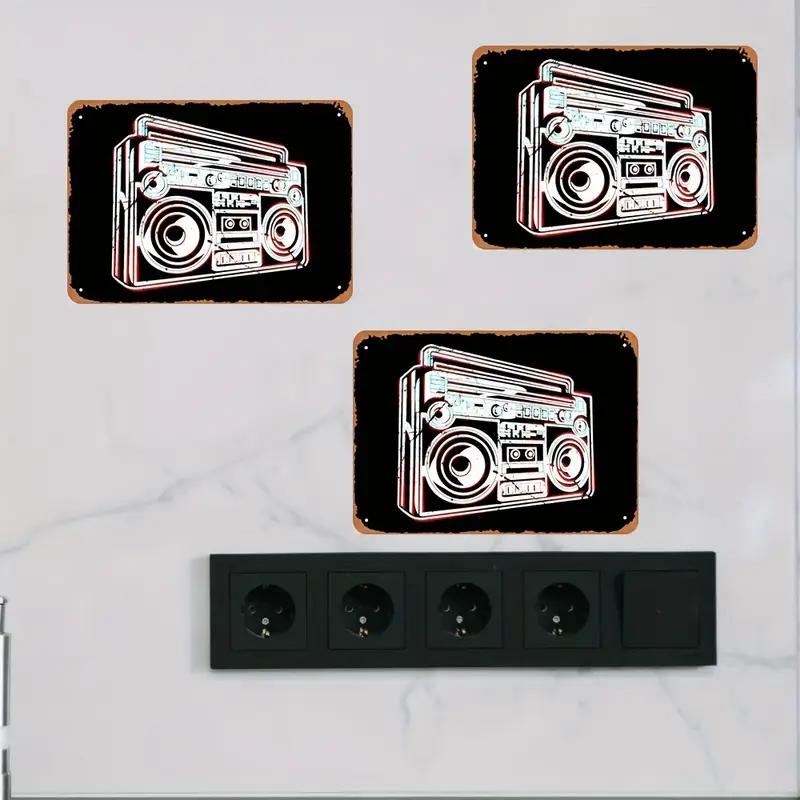The image depicts a marble-colored platform featuring three squares, each containing an illustration of a vintage boombox. These boomboxes, which appear to be either etched or stickered, are rendered in black and white and exhibit a slightly frayed or worn appearance. Each boombox displays classic features such as a tape deck, AM-FM radio, four speakers, and handles, and appears to be etched in an antique brass style. Below these squares lies a black rectangle with four recesses, which might represent musical connections or European plugs for electric purposes. The overall arrangement presents a nostalgic motif of old radios set against a sophisticated marble-like background.